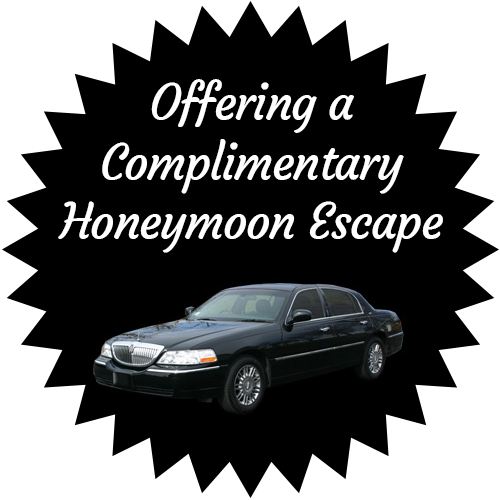On a pristine white background, the image prominently features a large black sun-shaped object, resembling a prize ribbon with numerous triangular protrusions encircling its perimeter. This black circular object dominates the center of the composition. At the top of this circle, stylish white text offers an enticing "complimentary honeymoon escape." Directly below the text, positioned near the bottom of the circle, is a sleek black four-door luxury sedan. The car, angled slightly to the left, boasts silver rims and black tires, complementing the overall monochromatic and silver aesthetic. The focus of the image, with its clean and striking design, suggests it could be an advertisement aimed at consumers, possibly for a car dealership or a hotel promotion.